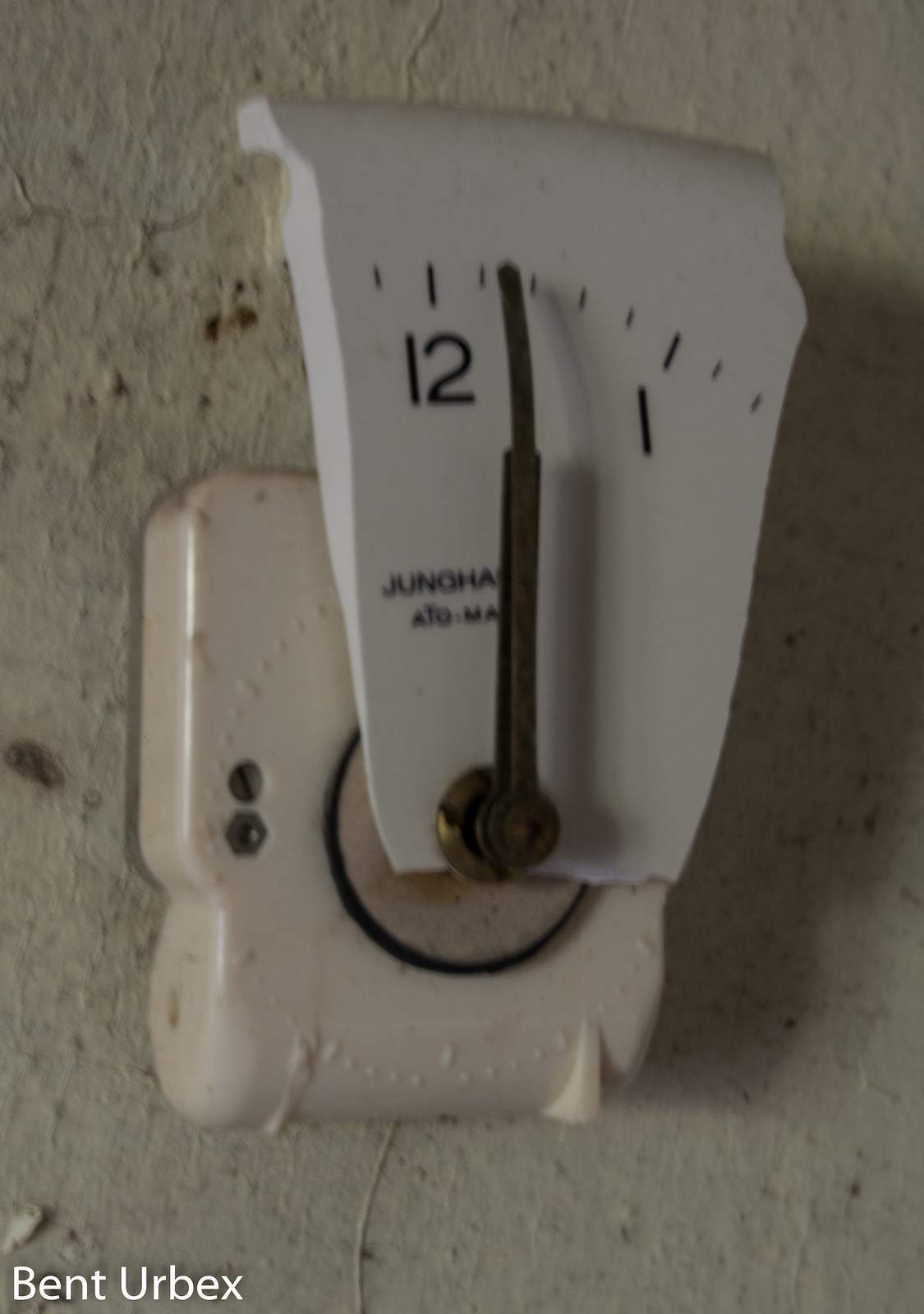This close-up image showcases a broken wall clock, with only a small section of the clock face visible, featuring the numbers 1 and 2. A clear plastic cover is positioned above this section. The clock's minute and hour hands are both stuck at the 12 o'clock position. Beneath the number 12, partially obscured by the clock hands, is the name "JUNGHA," with an additional letter hidden. Directly below this name, the text "ATO-MA" is partially visible, with the final letter obscured by the clock hands. The clock's motor remains intact and attached to the wall.